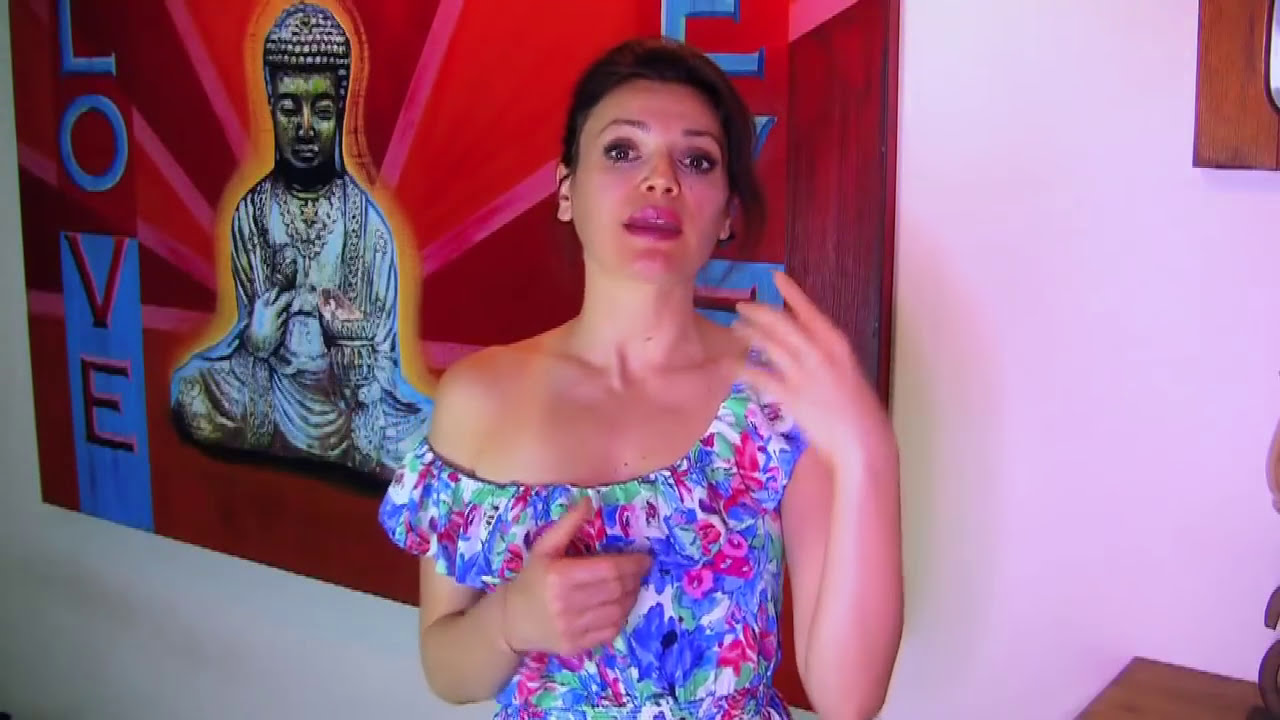The photograph features an Indian woman standing at the center of the frame, captured from the waist up. She has dark brown hair tied back and gazes directly into the camera with her mouth slightly open. She is wearing a vibrant, sleeveless floral dress with blue, green, white, and pink flowers, leaving her right shoulder bare. Her left hand is raised with fingers extended upward, and her right hand rests on her chest. The background includes a white wall adorned with several wall hangings. Prominently behind her is a large wooden art piece that displays the word "LOVE" in big blue and red letters, and part of a Buddha statue emitting light pink rays. In the lower right-hand corner, a wooden table is visible. The setting has a mix of wooden furniture, potentially indicating it could be a cozy home or a tastefully decorated business space.